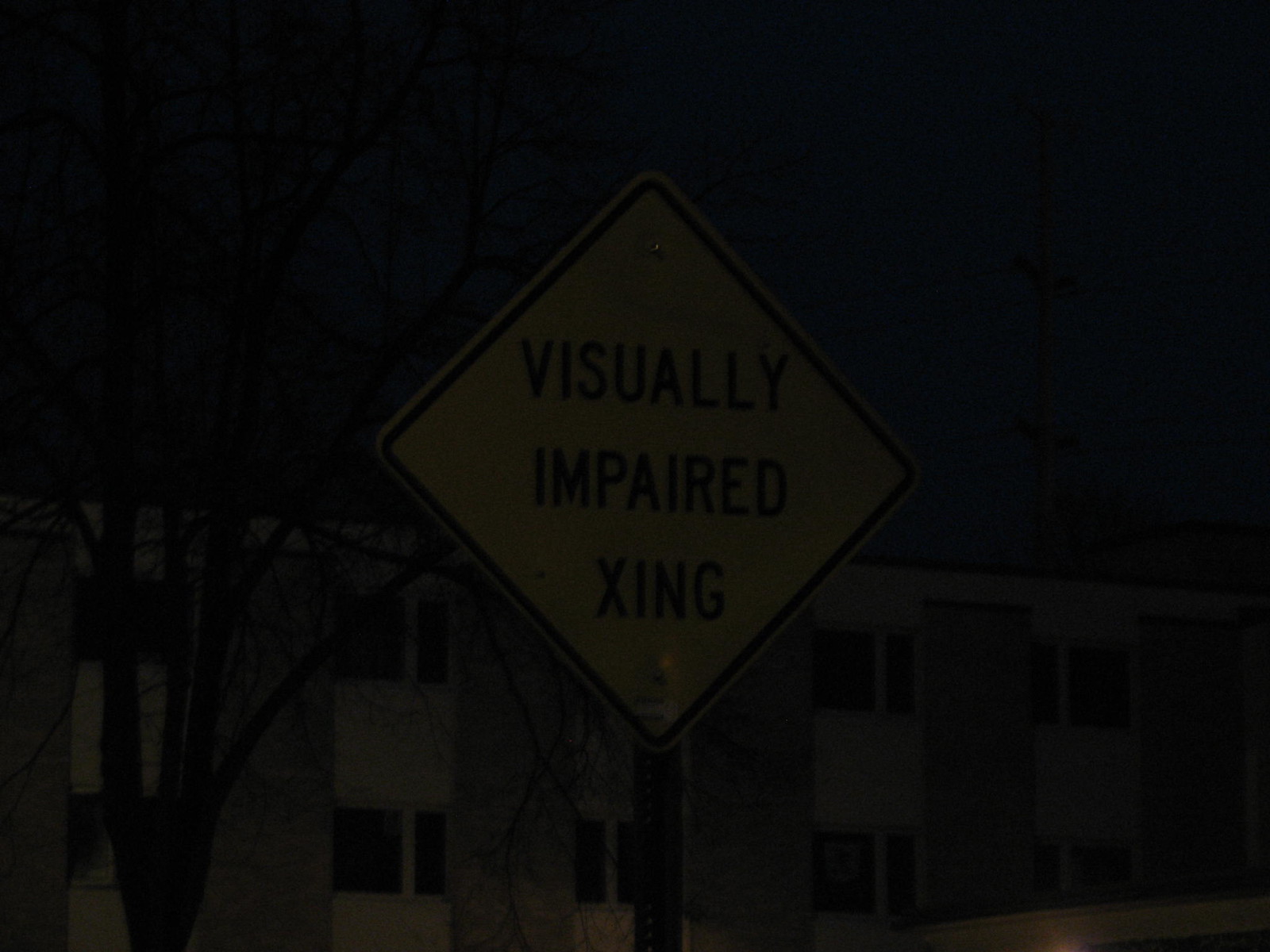A nighttime photograph captures a dimly-lit urban scene dominated by a diamond-shaped street sign at its center. The sign, likely yellow but appearing much darker due to the ambient darkness, features a thick black border and prominently displays bold, capitalized text reading "VISUALLY IMPAIRED X-ING." The sign is mounted on a pole, standing as a sentinel in the nocturnal landscape. Behind the sign, the silhouette of an apartment building looms, its darkened windows reflecting no light, framed by stone elements with a brownish hue. On the left side, a tree, seemingly lifeless with its barren branches, adds to the somber mood. To the right, partially obscured by the building, a tall power line pole stretches skyward, its lines faintly visible against the night sky. The overall composition evokes a sense of quiet solitude and urban decay.